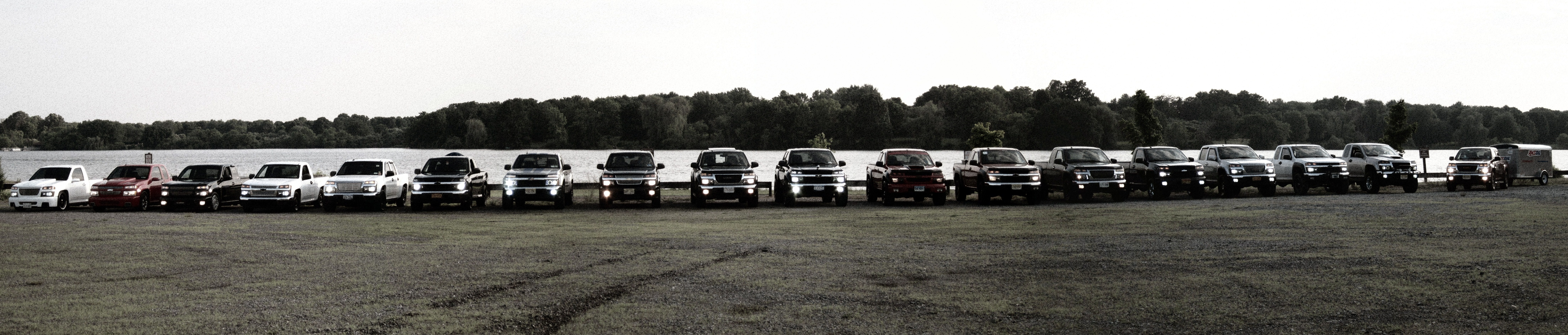This image is a panoramic grayscale photograph showcasing approximately 18 pickup trucks parked parallel to each other in front of a calm body of water. The trucks, lined up side by side in a gravel lot, have their headlights and windshields facing the viewer. A few of the trucks have their headlights on, while others do not. The truck on the far right-hand side is notably pulling a trailer. Behind the trucks, there is a still body of water, likely a large creek or an arm of a lake, that appears bright due to the black and white effect of the photo. In the background, a low hill covered with rows of trees stretches across the width of the image, beneath a hazy, overcast sky that lacks distinct cloud formations. The trucks are mostly dark in color, with a few white ones visible, contributing to the overall monochromatic scene that suggests an organized, perhaps promotional setup. The grassy area in front of the trucks is neatly trimmed, with visible patches where the grass is less green.